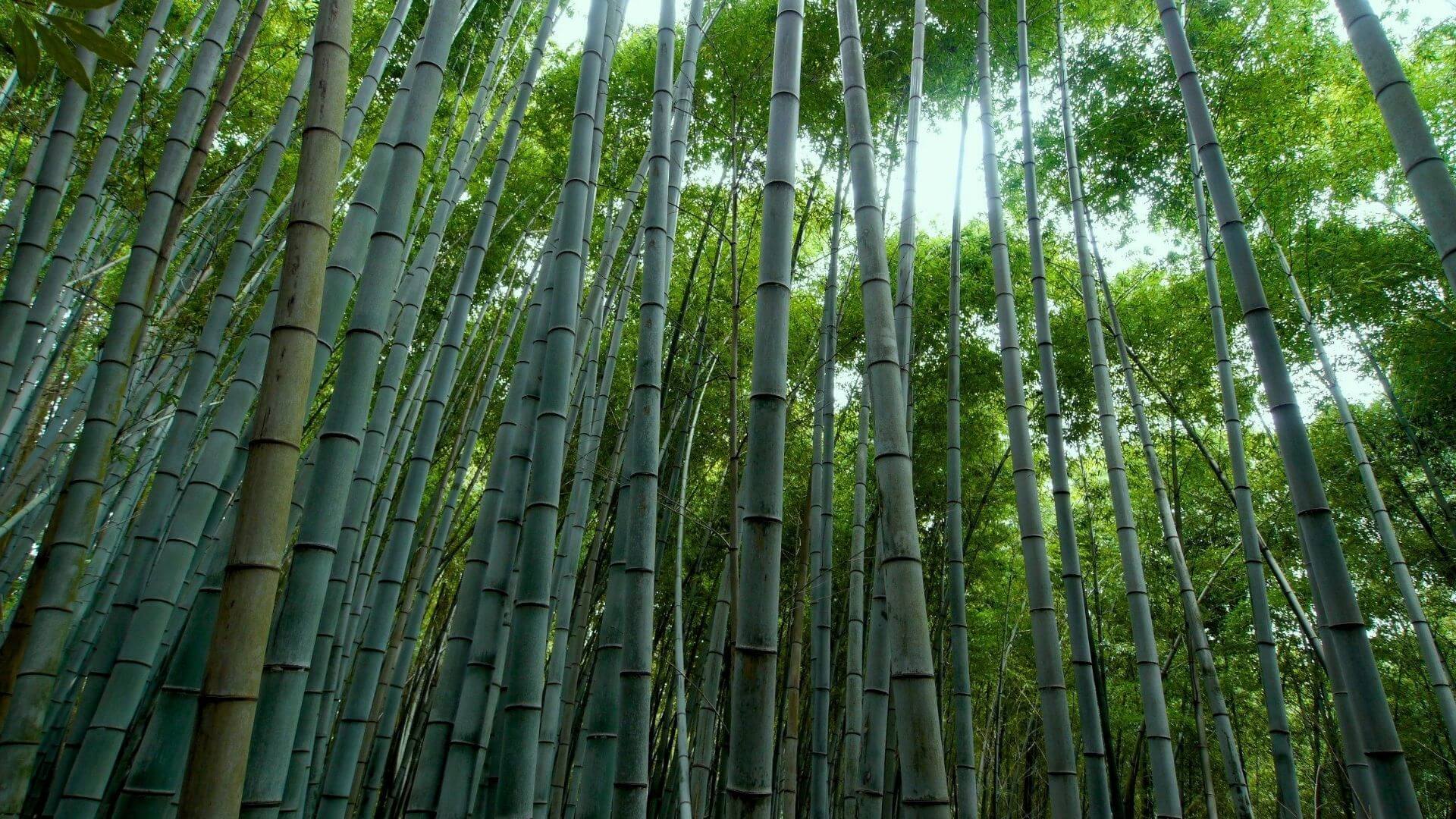This color photograph captures the interior of a densely packed bamboo forest, taken during the day with sunlight streaming through the canopy. From the perspective of someone standing amidst the trees, the viewer sees a thick stand of tall, thin, and uniformly shaped bamboo stalks, their trunks predominantly a medium shade of gray-green. Notably, on the left side of the image, a singular bamboo trunk stands out with a brownish hue. The bamboo stalks are tightly packed, creating a lush and immersive environment, though the density appears slightly less towards the right. Leafy green vegetation tops the bamboo, adding to the lushness, and through the gaps between the bamboo and leaves, patches of bright light indicate a sunny, possibly overcast sky. Despite the dense foliage, the brightness illuminates the forest floor, providing a clear and detailed view of this serene and verdant setting.